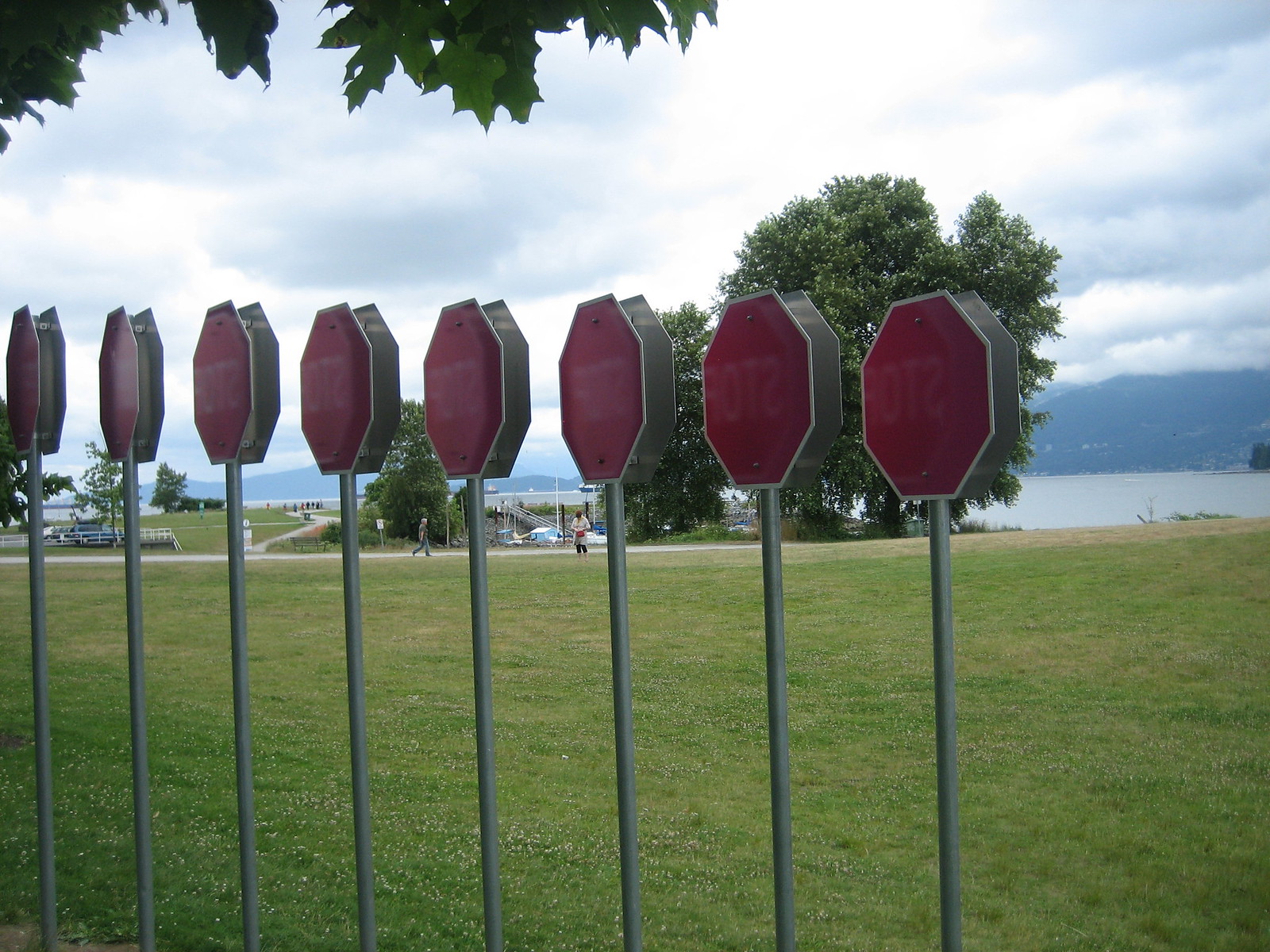The image presents a slightly angled view of eight red octagonal signs arranged side by side on stakes, resembling stop signs, though their white "STOP" lettering appears faded or rubbed off, making it difficult to discern. These signs are situated in the forefront of a spacious green field or park, under an overcast sky blending white with greyish-blue clouds. In the upper left corner, tree foliage is visible, while farther in the background, a serene bluish mountain range and a body of water create a distant horizon. Scattered across the grassy area, a couple of paths interweave, and one can also spot some tiny cars. Closer to the foreground, a few indistinct figures walk along the pathways, hinting at casual, recreational activity. Overall, the scene evokes the tranquility of a park, possibly near a marina, subtly hinting at its natural beauty and peaceful ambiance.